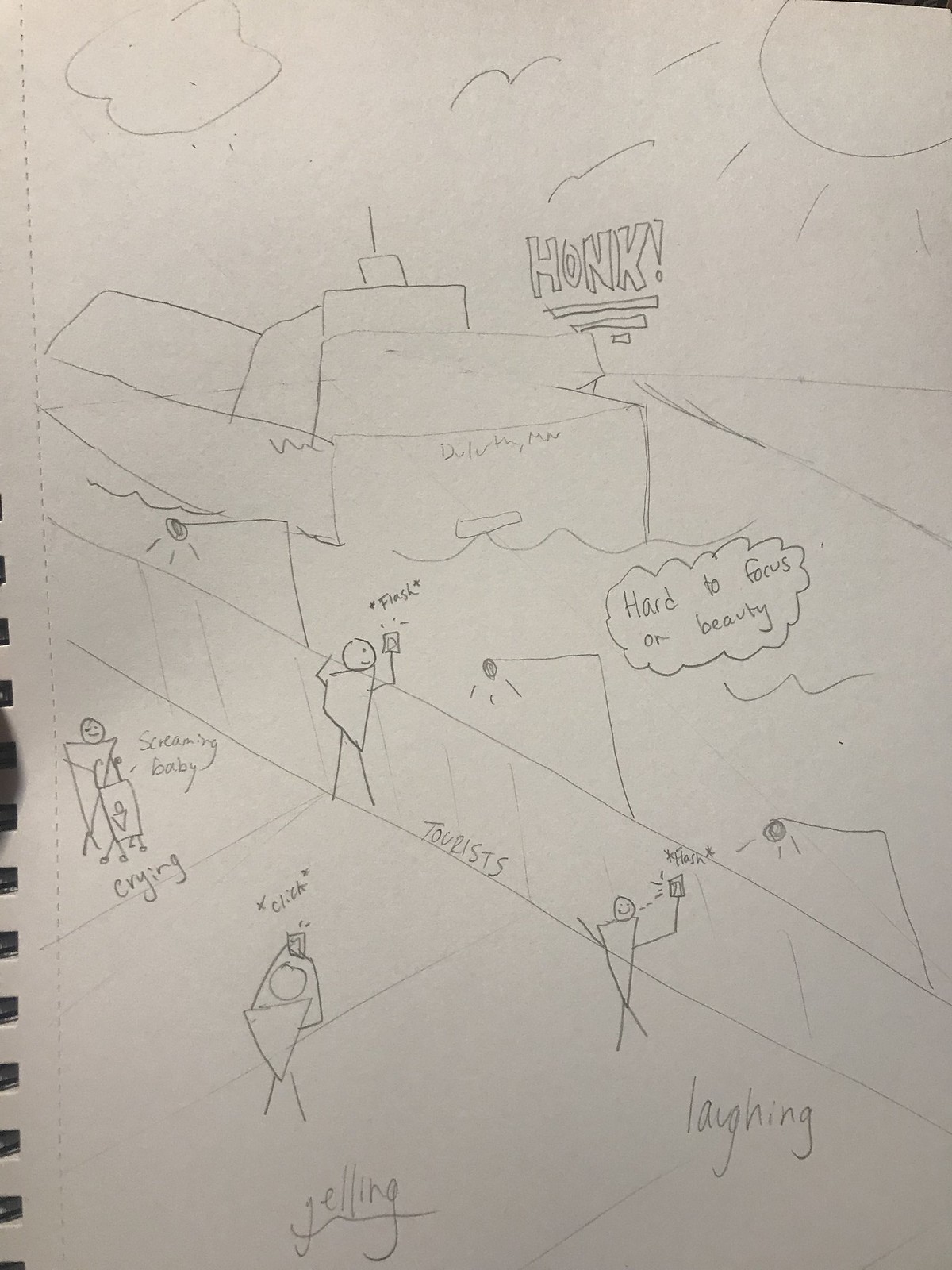This photograph captures a simple, pencil-drawn artwork on a piece of solid white notebook paper with a visible spiral binding on the left side and perforated edges. The unlined paper serves as a canvas for a straightforward stick-figure sketch depicting a whimsical scene by the marina. Central to the image is a stick-figure boat, labeled with "DULUTH MONTANA" on its stern and the word "HOG" prominently written in large capital letters nearby. A thought bubble emanates from the central part of the drawing, poignantly expressing, "HARD TO FOCUS ON BEAUTY."

Adjacent to the boat is what appears to be a marina wall, adorned with several stick-figure tourists. Detailed annotations within the drawing identify these figures: one holds a CRYING SCREAMING BABY, aptly labeled, while another snaps a photograph with a "CLICK" caption. Yet another tourist captures a selfie, denoted by the word "FLASH." The chaotic ambiance is further emphasized by the phrase "YELLING AND LAUGHING" scrawled at the bottom of the scene. The artwork, though simplistic in its execution, thoughtfully conveys a layered narrative of distraction and chaos, subtly juxtaposed against the serenity of the marina setting.